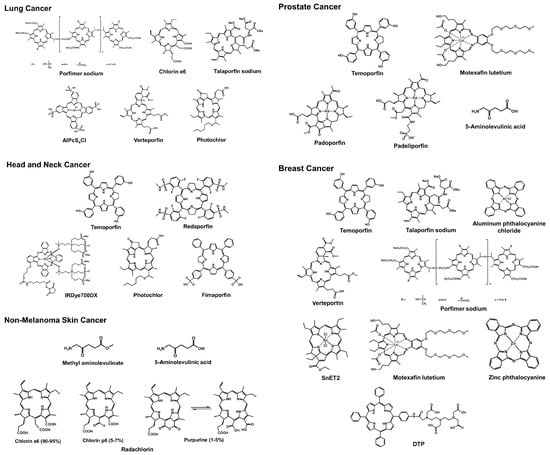The image features a minimalist white background with black text and clustered illustrations of molecular structures. In the top left corner, the title "Lung Cancer" is displayed, accompanied by a dense cluster of chemical diagrams, including one labeled "Chlorine E6." To its immediate right is another group of molecular figures under the heading "Prostate Cancer."

Below these, the next row contains two more clusters. On the left, "Head and Neck Cancer" is denoted, with its corresponding molecular maps. Directly next to it, on the right, is a cluster labeled "Breast Cancer," showing detailed chemical bonds and their respective names.

At the bottom left of the image, the final cluster is labeled "Non-Melanoma Skin Cancer," again featuring intricate diagrams of molecular structures, each clearly labeled. The chemical maps illustrate various bonds and configurations, providing a scientific visual representation for each type of cancer listed.